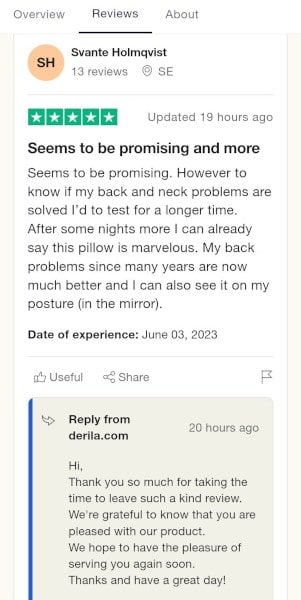A detailed, cleaned-up version of the original caption could be:

---

The image displays a smartphone screen showing a review page. At the top, three tabs are visible: "Overview," "Reviews," and "About." The "Reviews" tab is highlighted with a black underline. Below, a review box features an orange circular icon with the initials "HS" next to the name "Savanti Holomquist," who has submitted 13 reviews. An icon representing location followed by "Southeast" is also visible.

To the left, there are five green boxes with white squares inside them, indicating a rating. Text next to this reads "Updated 19 Hours Ago." The review's title, "Seems to be Promising and More," is in bold font, followed by a detailed review in lighter font: "Seems to be promising. However, to know if my back and neck problems are solved, I test for a longer time. After some nights more, I can already say this pillow is marvelous. My back problems since many years are now much better, and I can also see it on my posture (In the Mirror)."

Below this, the "Date of Experience" is in bold, followed by "June 3rd, 2023" in lighter font. There are buttons for "Useful," "Share," and a flag icon to report the review. A gray box underneath indicates that someone has replied to this review.

---

This version is more structured and detailed, making it easier to visualize the described image.